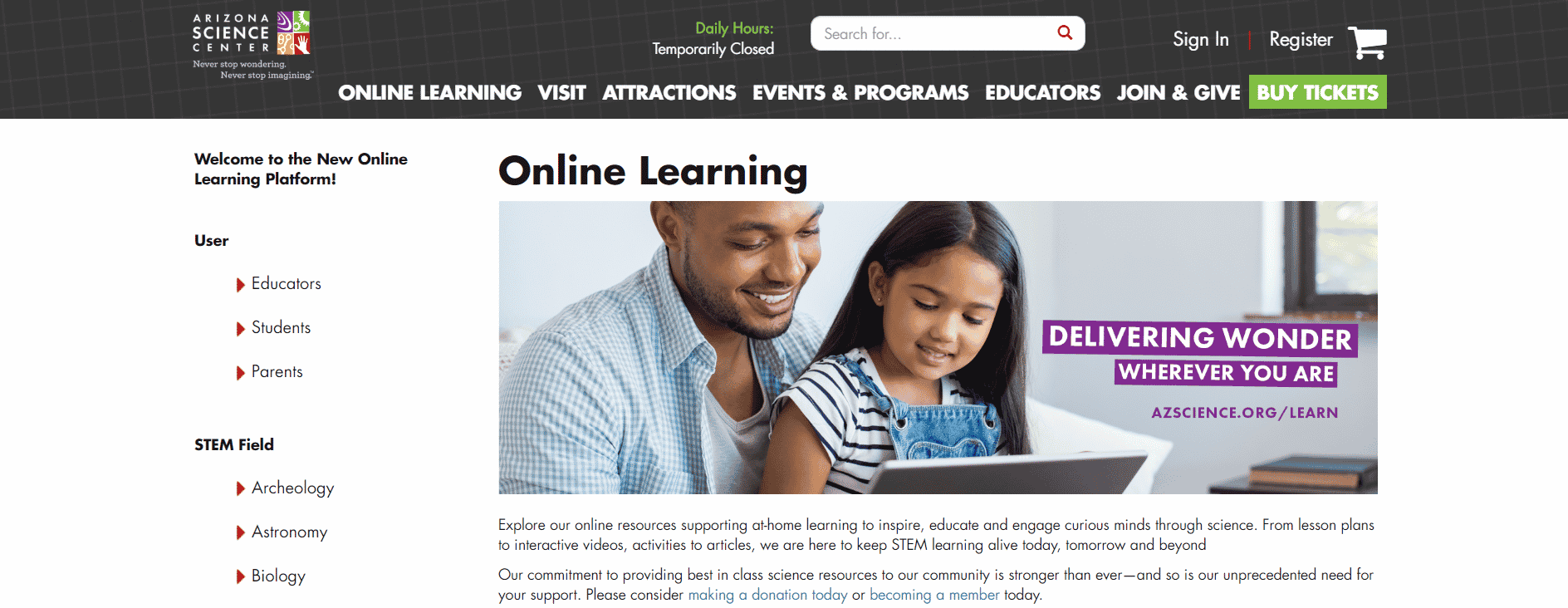**Screenshot of Arizona Science Center's Online Platform**

The image appears to be a screenshot of the Arizona Science Center's online platform. The layout is framed by a thick black border at the top, containing the center's logo and various navigation options. 

**Top Black Border:**
- **Logo:** On the left side, the Arizona Science Center's logo is displayed, which is a square divided into four smaller squares colored gold, red, green, and purple. These geometric shapes collectively form the silhouette of a hand.
- **Slogan:** Beneath the logo is the slogan, "Never Stop Wondering, Never Stop Imagining," written in white text.
- **Center Section:** Next to the logo, in the center of the border, it states "Daily Hours" in green text, followed by "Temporarily Closed" in white text.
- **Search and Account Options:** On the right side, there is a search box, a sign-in button, and a cart icon.
- **Main Menu:** The menu includes options like Online, Learn and Visit, Attractions, Events and Programs, Educators, and Join and Give, all in white text. There is also a green button labeled "Buy Tickets."

**Left Column:**
- **Header:** "Welcome to the New Online Learning Platform" is prominently displayed in bold black text.
- **Dropdown Menus:** There are two sections with dropdown menus:
  - **User Section:** Includes options for Educators, Students, and Parents.
  - **STEM Field Section:** Lists Archaeology, Astronomy, and Biology.

**Main Content:**
- **Central Photo:** The central part of the page features a large photo of a father and child looking at a laptop together.
- **Overlay Text:** The text on the photo reads “Online Learning” with a tagline “Delivering Wonder Wherever You Are,” followed by the URL "azscience.org/learn."
- **Subtext:** Below the image, there's a brief text encouraging visitors to explore the online resources available.

This screenshot serves as a gateway to the various educational offerings and online resources that the Arizona Science Center provides, emphasizing accessibility and engagement in science education from anywhere.